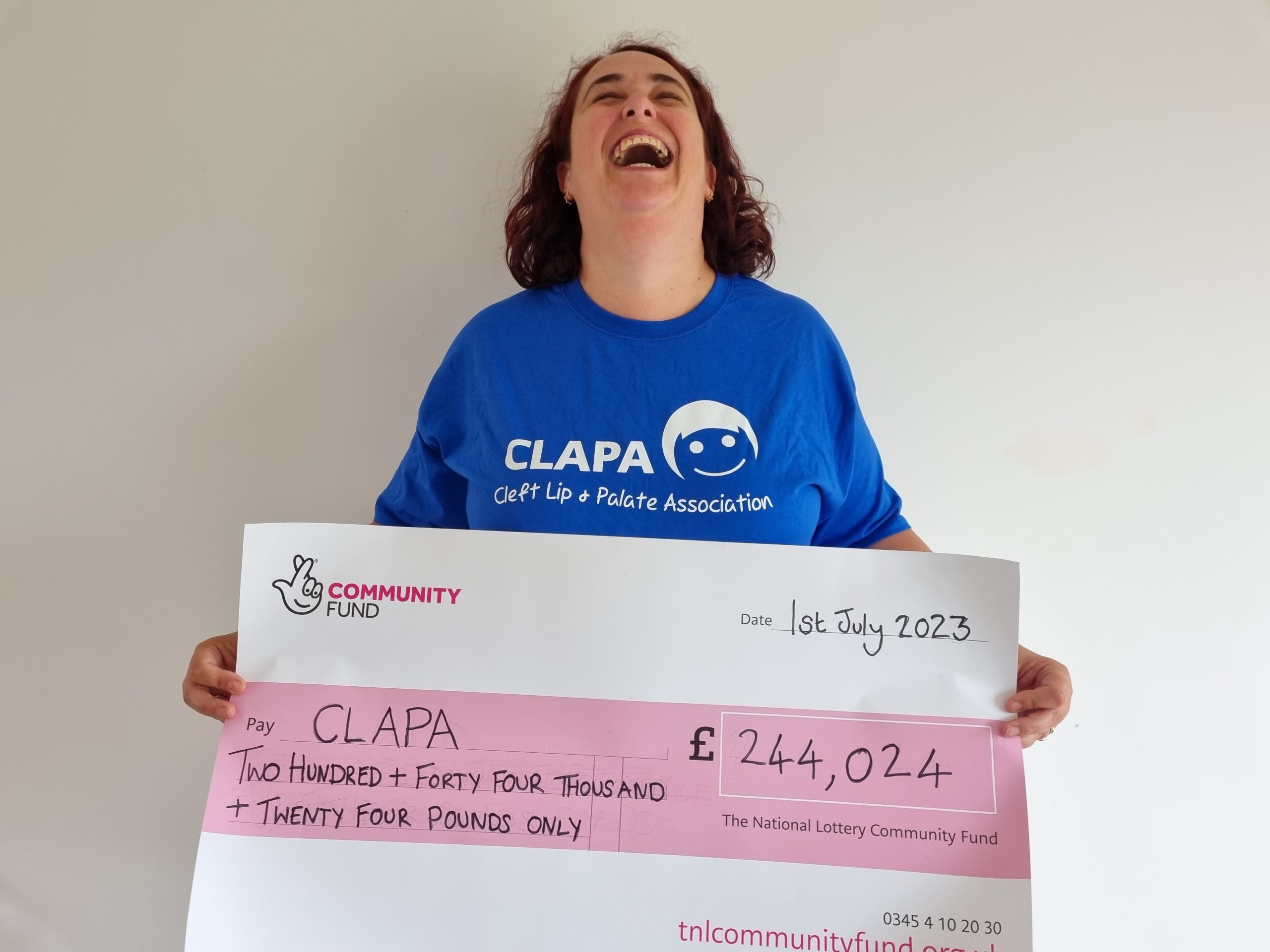A woman with reddish-brown, shoulder-length curly hair, wearing a blue t-shirt that reads "CLAPA: Cleft Lip and Palate Association," stands in front of a gray backdrop. She is joyfully smiling and laughing with her mouth open wide. She holds up a large ceremonial check displaying the National Lottery Community Fund logo. The check is dated 1st July 2023, made out to CLAPA for the amount of £244,024. It also includes the organization's name, "Community Fund," and the website "tnlcommunityfund.org". In the lower section of the check, the amount is repeated as "244,024 pounds only," and a check number "03454102030" is visible. The woman’s expression of happiness is palpable, reflecting the significance of the donation to the organization she represents.